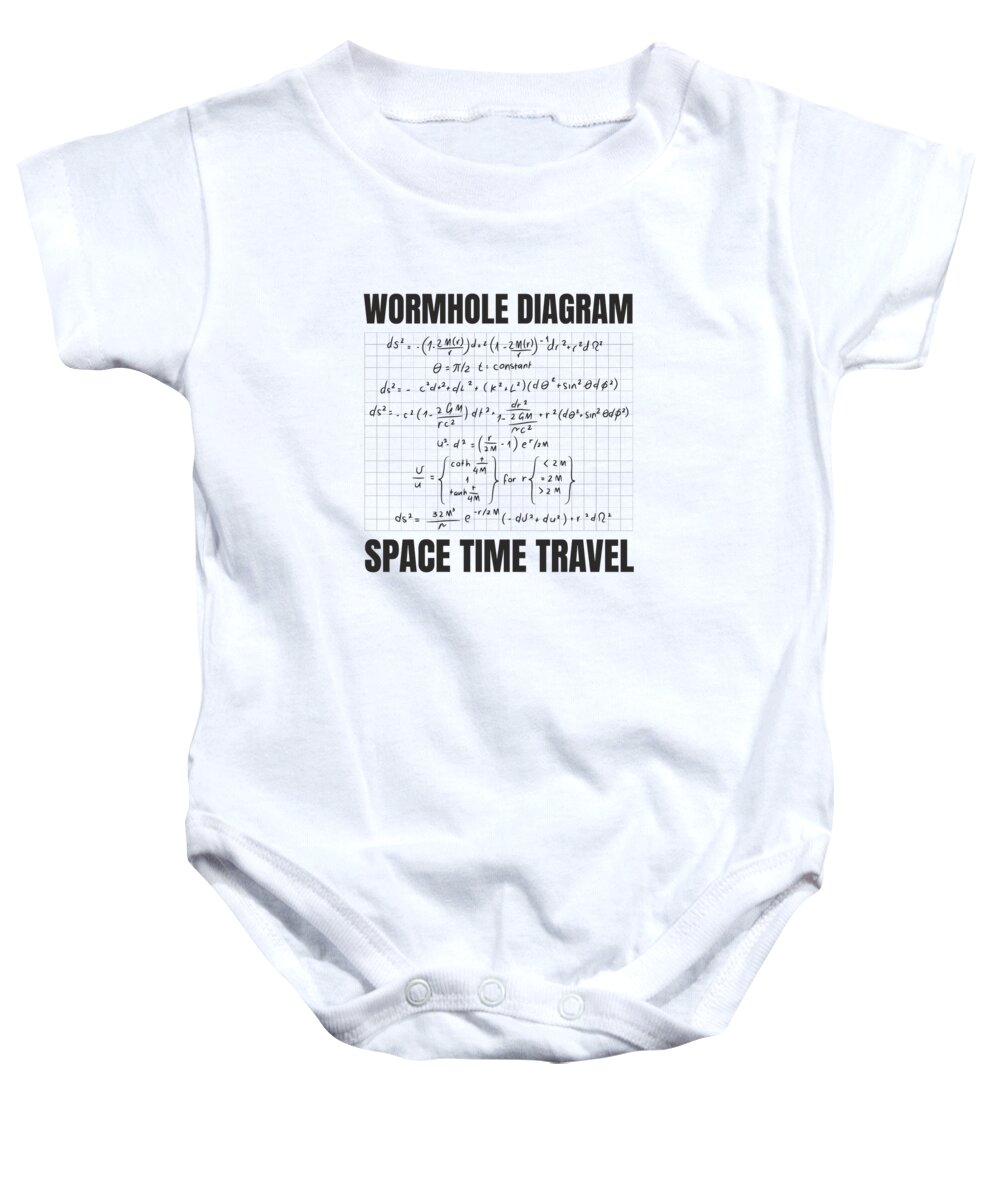This image features a white baby onesie with short sleeves, lying on a white background with slight wrinkles giving a light blue hue to the folds. The onesie has three snap buttons at the crotch area for easy diaper changes. The front of the onesie prominently displays a design centered around a square of graph paper. Above this square, in bold black text, are the words "WORMHOLE DIAGRAM." The graph paper section is filled with multiple lines of equations and calculations related to the wormhole diagram, including some expressions with brackets. Below the graph paper, the phrase "SPACE-TIME TRAVEL" is written in large, uppercase black letters. The onesie is positioned facing forward in the image, giving a clear view of the detailed design.